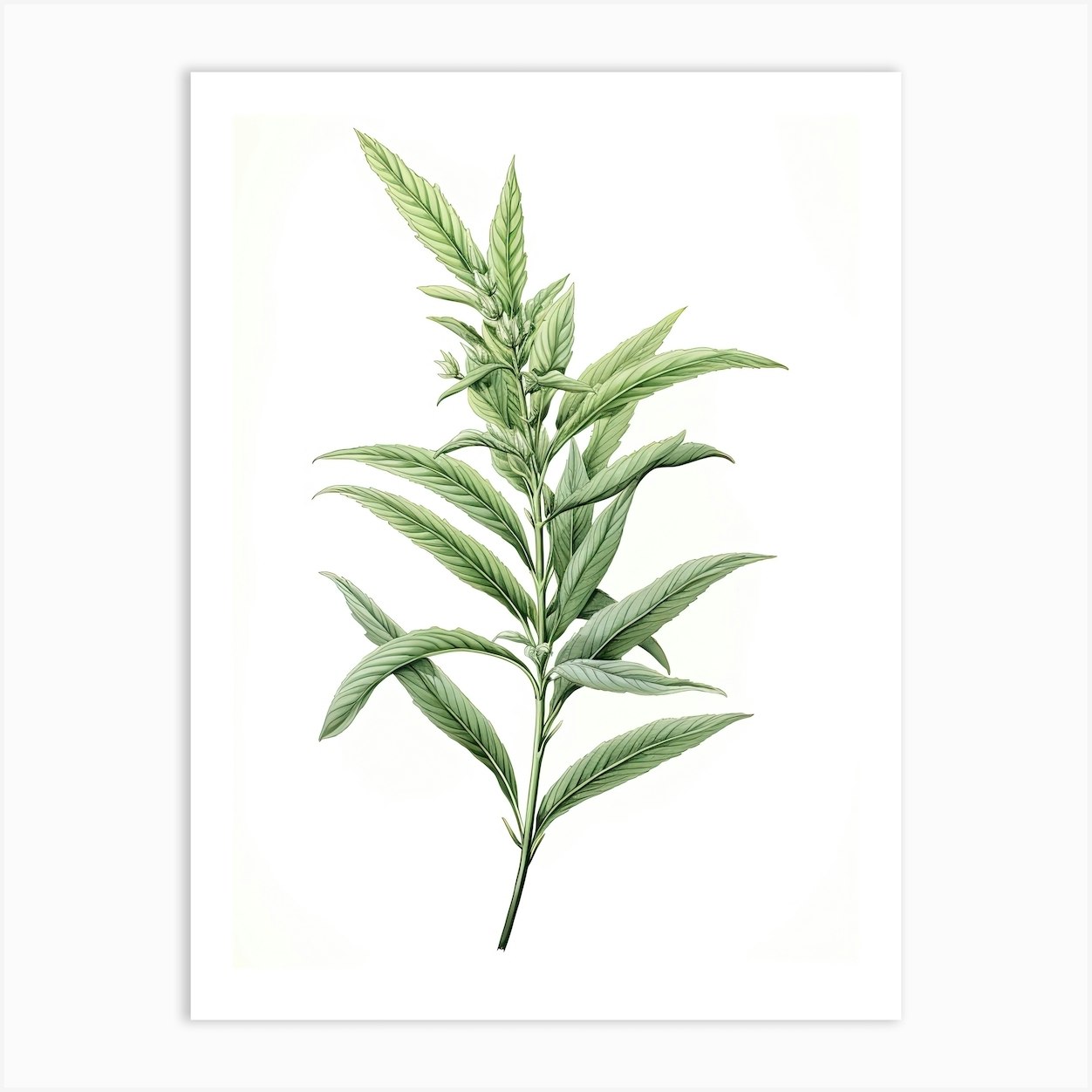This illustration features a single, green plant set against a completely white background. The plant's slender, long leaves, which taper to a point at the tips, grow directly from a central stem in a uniform green color with dark shadows or lines that lend depth to the image. The leaves are arranged symmetrically with two extending from each section of the stem, alternating left and right, with some sections also featuring a middle leaf. Near the top of the plant, the leaves cluster together more densely. Among the leaves, some buds are visible, hinting at the potential of flowering, with a resemblance to wheat heads but more likely representing unopened blossoms. The entire plant's simplicity and repetitive structure dominate the white canvas, making it the focal point of the artwork.